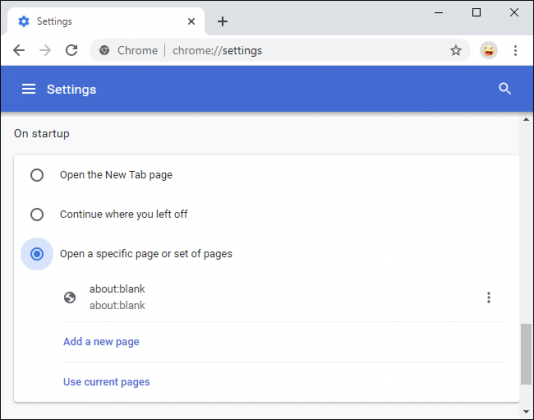In this detailed screenshot of a computer screen, we observe an open browser window with various navigational and operational elements visible. 

At the top right corner, there are standard window control icons: a solid line for minimizing, a square for maximizing, and an 'X' for closing the window. On the left-hand side, there is a visible tab featuring a blue gear icon accompanied by the word "Settings." Adjacent to this tab, there is an 'X' icon designed to close the tab.

Directly below the tab bar, a navigational toolbar includes a selectable left arrow, a non-selectable (grayed-out) right arrow, and a circular arrow for reloading the page. This toolbar also displays the URL "chrome://settings" next to the word "Chrome" separated by a vertical bar. To the right of the address bar, there is a star icon for adding the page to favorites (which is not selected), an emoticon icon resembling a smiley face, and a vertical three-dot menu icon.

Beneath this toolbar, a prominent blue banner reads "Settings," featuring three horizontal lines on the left to access settings choices and a magnifying glass icon on the far right for searching within the settings.

Further down, the page transitions into a light blue section titled "On Startup," followed by a large white box containing three startup options. These options include:
1. "Open the New Tab page."
2. "Continue where you left off."
3. "Open a specific page or set of pages," with the third option currently selected.

Within this selected option, two items labeled "about:blank" are listed, each with an accompanying globe icon symbolizing a webpage. Below these entries, there is a blue link titled "Add a new page," and an option labeled "Use current pages."

Overall, the image meticulously showcases the browser settings interface in a detailed and intuitive layout.